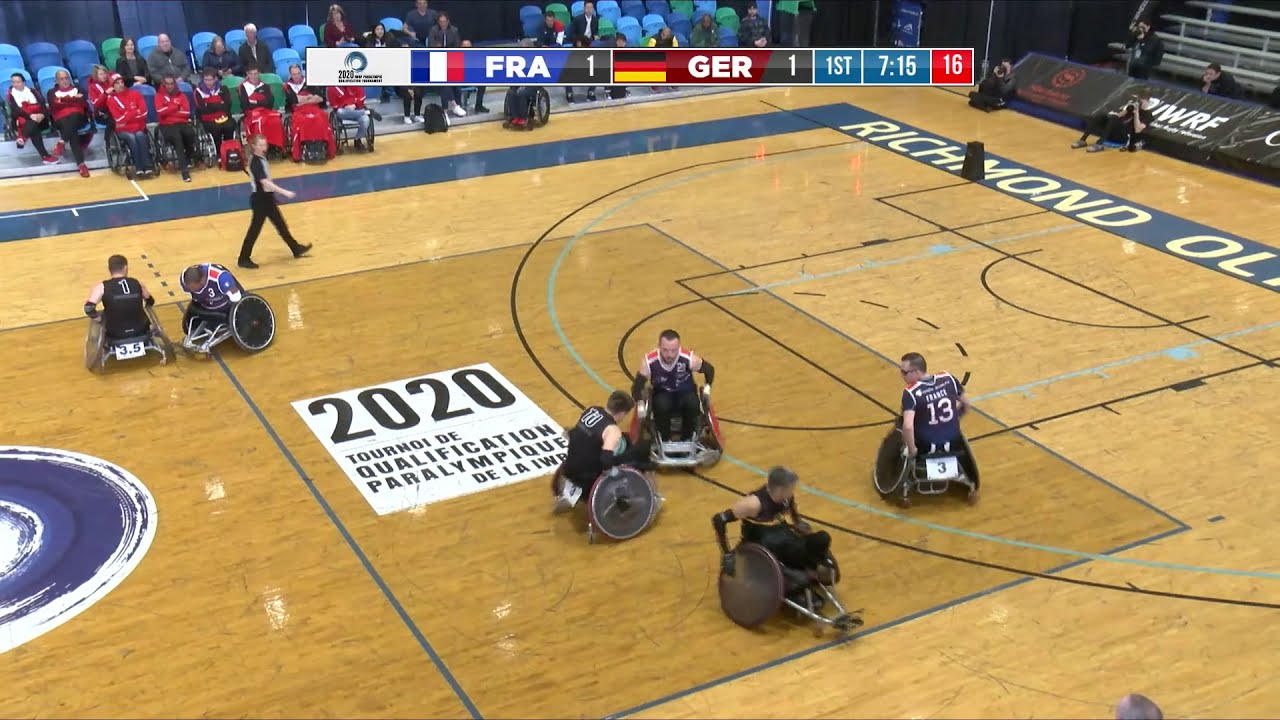The image, taken indoors, captures a wheelchair sports competition held on a basketball court. The arena floor prominently displays a large white sticker with text partially in French, reading, "2020 Tournoi de Qualification Paralympique de la IWA." Above the court, the scoreboard indicates a match between France (FRA1) and Germany (GER1), with the score standing at 1-1 during the first quarter, with 7 minutes and 15 seconds remaining. In the middle of the court, six male athletes in wheelchairs are actively engaged, wearing jerseys, with one of the players notably missing arms and using nubs. A referee or coach can be seen walking around, and an audience sits on the sidelines in blue chairs, attentively watching the game. The right side of the court features "Richmond OL," adding to the competition's international atmosphere.